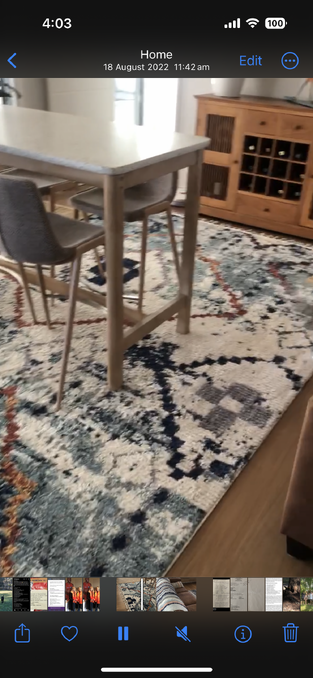The image depicts a screenshot taken on a phone. At the top, a black banner displays the time "4:03" in white on the upper left corner, accompanied by icons for battery, network, and signal strength on the upper right. The main image showcases a multicolored area rug primarily in cream, featuring accents of navy, rust, and light green in geometric patterns. Towards the back, a wooden wine cabinet is visible, equipped with a cabinet door on the left which incorporates two glass-panelled sections. Atop the cabinet, there is an indistinguishable white planter, partially cropped out of view. Centrally positioned on the rug is a table set with two chairs. The table has brown legs and a white tabletop, while the chairs feature metal legs and plastic bucket seats. At the bottom of the screenshot, the phone's gallery interface is partially visible, displaying thumbnails of other images. A black banner at the very bottom contains icons for sharing, liking, pausing, adjusting sound, viewing information, and deleting.